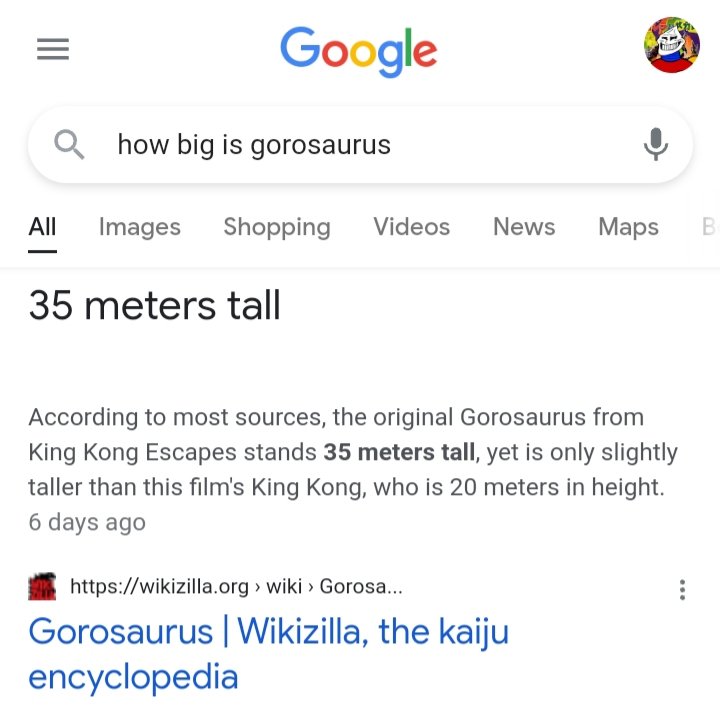In the image, we see a Google search page prominently displayed. At the top right of the screen, there's a circular profile picture featuring the iconic troll face, which is white, set against a vibrant background with splashes of yellow, red, green, orange, and purple. The person in the picture is also wearing a red shirt. Dominating the interface at the top center is the Google logo, colored in the familiar sequence of blue, red, yellow, blue, green, and red. 

On the top left, a light gray hamburger menu icon is visible. Just beneath the Google logo is the search bar. The query inside it reads, "how big is a gorosaurus," with a magnifying glass icon on the left side of the bar and a microphone icon on the far right. 

Directly below the search bar, there are multiple categories listed: 'All' is selected, highlighted in a darker black with a black underline, followed by 'Images,' 'Videos,' 'News,' and 'Maps,' each written in a lighter gray. 

Further down, the top search result is displayed, stating, "35 meters tall." The accompanying description reads, "According to more sources, the original Gorosaurus from King Kong Escapes stands 35 meters tall, yet is only slightly taller than this film's King Kong, who is only 20 meters in height."